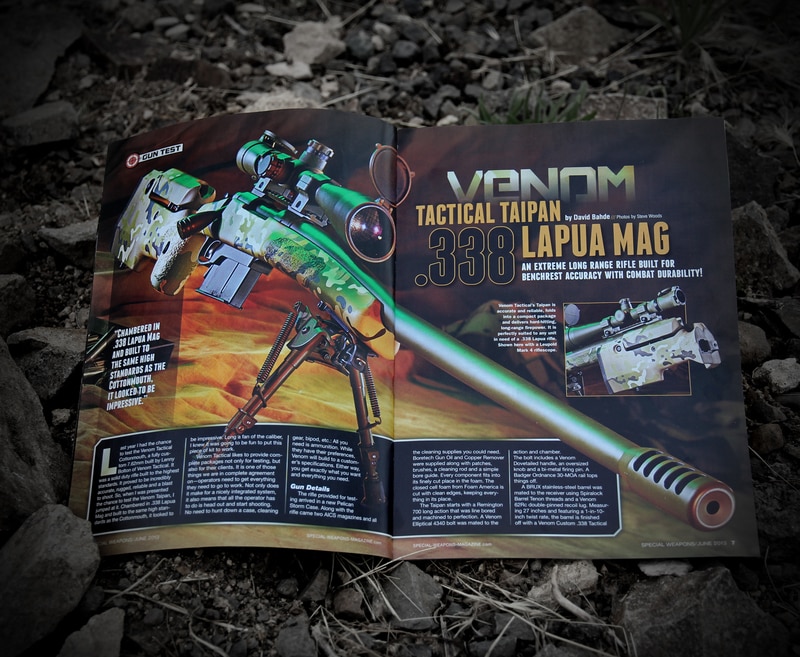The image depicts a rifle magazine spread open on a ground littered with small rocks, stones, pine needles, and sprigs of grass, evoking a natural, outdoor setting. The magazine pages showcase a detailed illustration of the Venom Tactical Taipan, a .338 Lapua Magnum rifle. The rifle, characterized by its long, gunmetal gray barrel tinged with greenish hues, is mounted on a tripod. It features a camouflage-patterned stock and a similarly hued scope. In the upper left corner of the spread, a red bullseye icon with a white tag labeled “Gun Test” is visible. The right-hand page includes a prominent inset detailing the trigger mechanism, while the text on both pages describes the rifle’s capabilities, emphasizing its extreme long-range accuracy and combat durability. The background is mostly black with white font, forming a rectangular text block spanning both pages, which reviews the rifle in detail. The rifle's name and specifications, "Venom Tactical Taipan .338 Lapua Mag," are prominently displayed at the top, with "Venom" in large letters and additional descriptive text and numbers underneath.